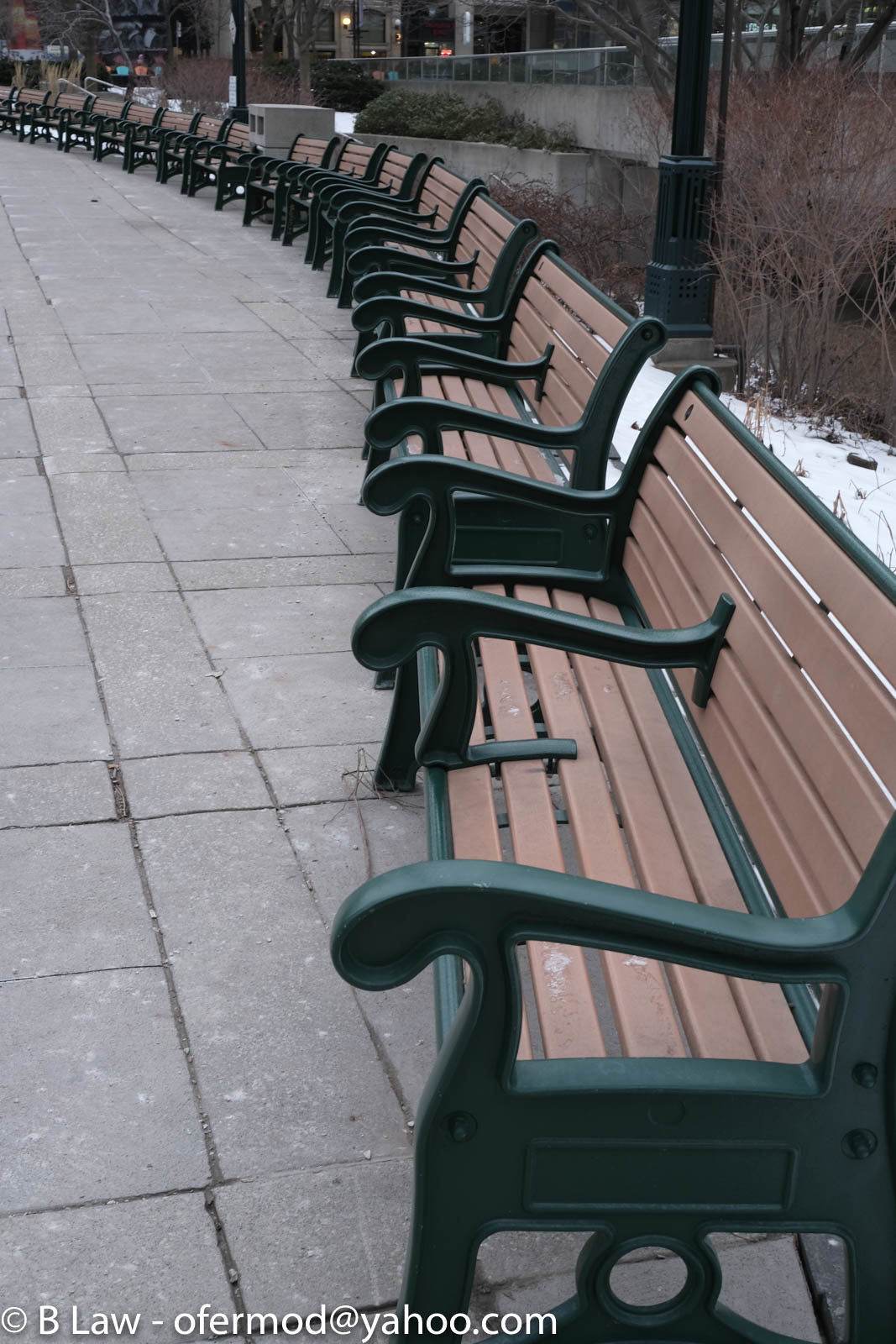The outdoor image features a long row of identical, well-maintained park benches aligned next to each other on a concrete walkway that has lines etched into it. Each bench is constructed with a black metal or hard plastic frame and adorned with tan or tannish-brown slats. The setting includes a large building in the background, flanked by green bushes, leafless branches, and patches of white that suggest snow, hinting at a winter scene. Central in the background is a distinctive round-topped light post with a glass segment near its concrete base. Notable details include a faint trace of bird droppings on the bench closest to the camera and the bottom edge of the image displaying a partial and unclear inscription, possibly 'B-Law'. The overall atmosphere appears cloudy, creating a subdued light.